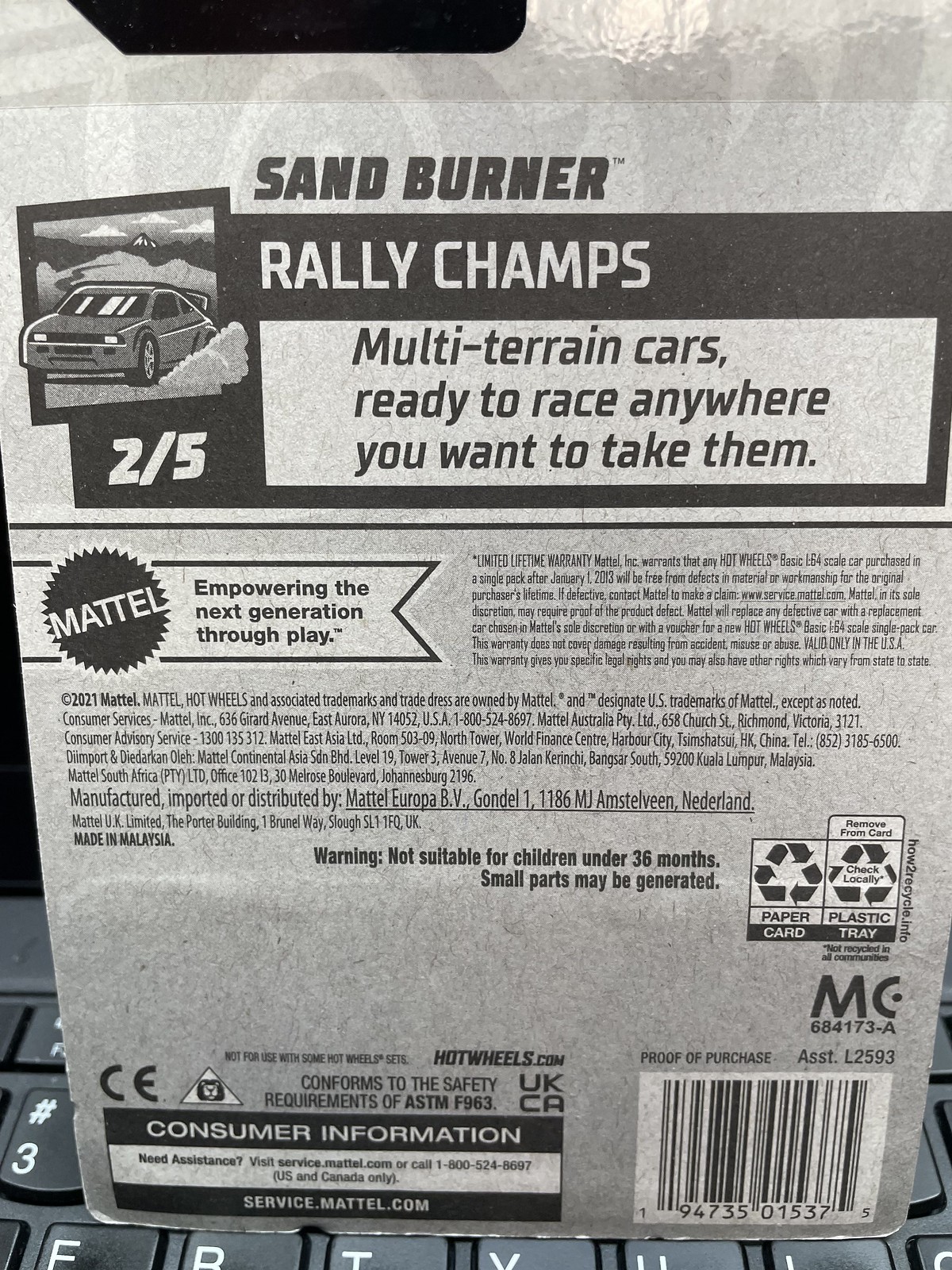This black-and-white photograph captures the back of a Mattel toy car package, specifically from the Sandburner Rally Champs series, described as multi-terrain cars ready to race anywhere you want to take them. In the upper left corner, there is a cartoon drawing of a race car labeled with "2/5," indicating it is the second model out of five in this series. Below this, the bold Mattel logo is prominently displayed, accompanied by their tagline, "Empowering the next generation through play." The lower part of the packaging carries a warning message stating that the toy is not suitable for children under 36 months due to small parts which may be generated. Additionally, it contains recycling instructions, consumer information, and a barcode—94735-01537—positioned in the bottom right corner. Visible in the background of the image is a computer keyboard, over which the packaging rests.